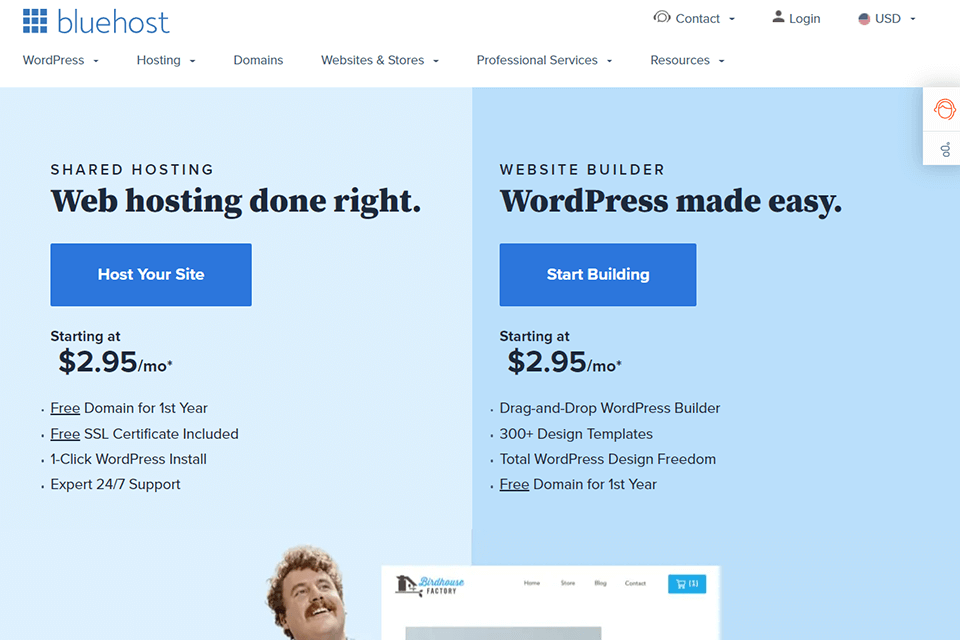Here is a more detailed and cleaned-up caption for the image described:

---

The image is divided into two distinct sections within a rectangular frame. The top portion features a blue box comprised of nine smaller squares, displaying the text "Bluehost" in white, followed by a white space. Adjacent to this are options labeled "Contact," "Login," and "NUSD." Beneath this, a navigation bar lists "WordPress," "Hosting," "Domains," "Websites & Stores," "Professional Services," and "Resources," each accompanied by a drop-down arrow.

The left half of the rectangle is shaded in a lighter blue and highlights the title "Shared Hosting - Web Hosting Done Right." Below this, a darker blue rectangle with the title "Host Your Site" details an offer starting at $2.95 per month. This offer includes features such as a free domain for the first year, a free SSL certificate, one-click WordPress installation, and expert 24/7 support.

Adjacent to this, another darker blue rectangle titled "Website Builder - WordPress Made Easy" invites users to "Start Building." The highlighted offer also starts at $2.95 per month and promotes a drag-and-drop WordPress builder, over 300 design templates, complete WordPress design freedom, and a free domain for the first year.

The bottom of the image features a joyful man looking upwards, capturing a sense of satisfaction. Adjacent to him, a white box contains the text "Factory" along with a shopping cart icon, suggesting e-commerce capabilities.

---